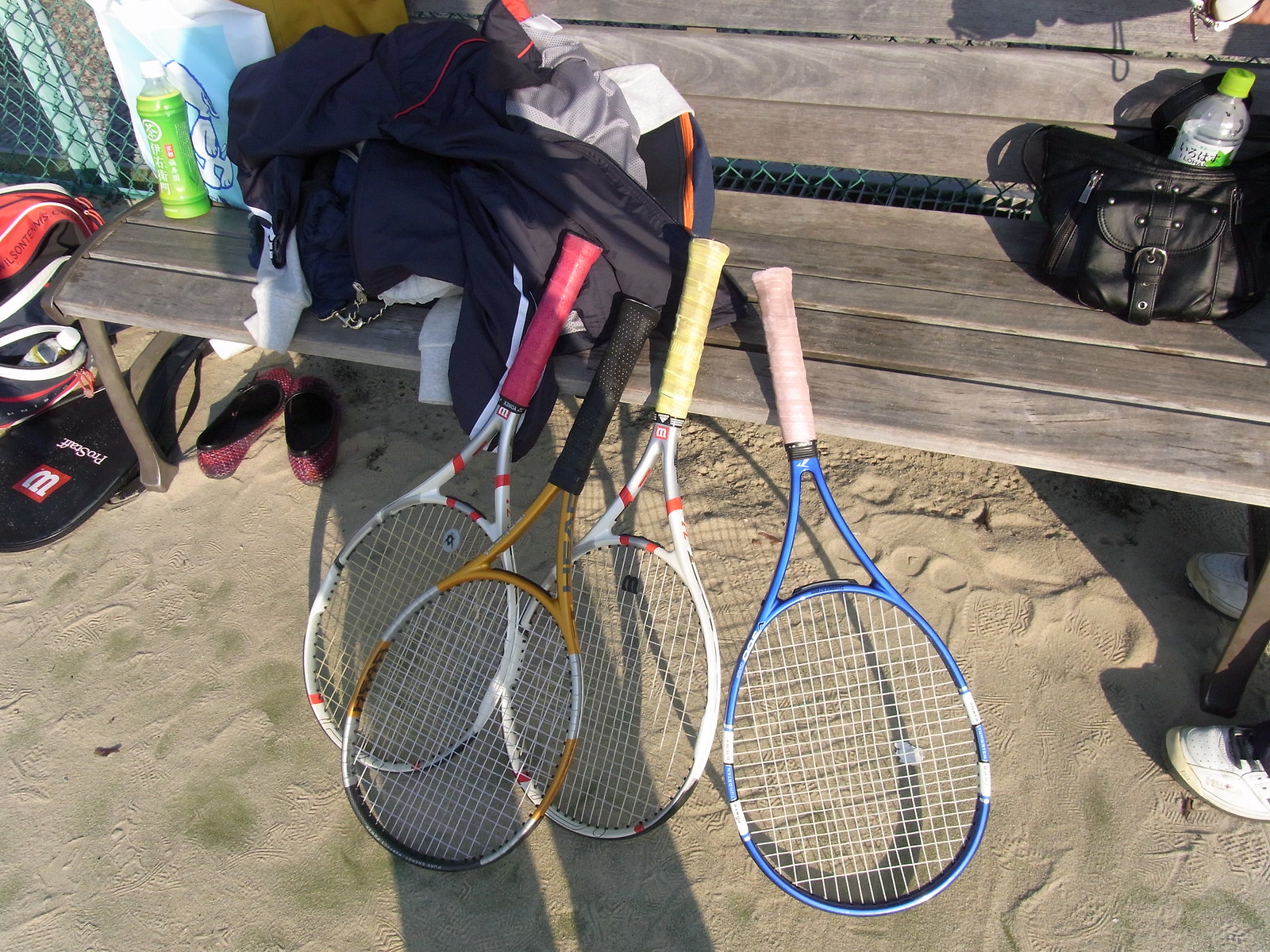The photograph captures an outdoor setting, likely a baseball field or stadium due to the sandy ground and presence of a chain-link fence typical of a baseball dugout. The focal point is a wooden bench in front of the fence, which is laden with various items. Four tennis rackets are prominently leaning against the bench; their handles display a palette of colors including white, red, blue, yellow, black, and pink. Atop the bench are several bags, including a black bag that might be a camera bag, along with a couple of bottled beverages—one with a green cap and a white-green label. A plastic sack featuring a Snoopy character is also visible. Scattered around and under the bench lie clothes, including a blue top, a white item, and possibly jackets. Two pairs of shoes can be seen, one pair white with black laces. Additional items, such as what seems to be a black and red garment or towel and a green bottle, add to the scene’s cluttered yet vivid detail.